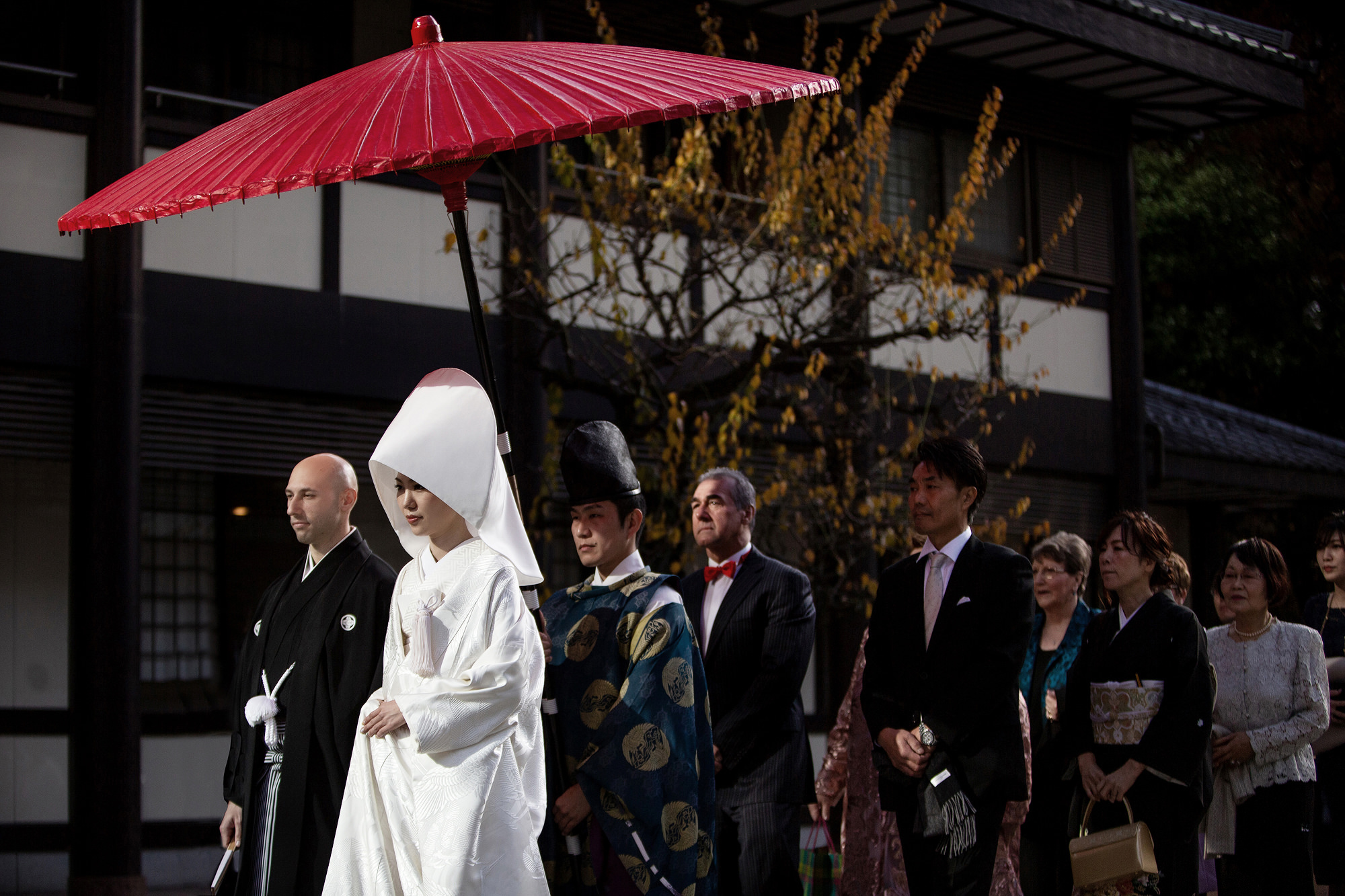The photograph depicts a traditional Japanese wedding ceremony held in front of a Japanese temple. Leading the procession is a woman clad in a white robe and a large white hood, symbolizing the bride. She walks under a decorative red umbrella held by someone to provide her shade. Beside her stands a man dressed in traditional Japanese attire consisting of a black robe and a white tie, likely the groom, holding something in his right hand. The groom is identified as bald and dressed formally. Accompanying the couple is another man similarly dressed in traditional Japanese clothing, possibly a ceremonial figure or family member. Following them are two rows of people, including individuals in tuxedos, further signifying the formal nature of the occasion. Among the procession are older men, likely the fathers of the bride and groom, wearing respectively traditional Japanese clothing and an Eastern-style tuxedo. The scene is rich with cultural elements, underscoring the solemnity and heritage of a traditional Japanese wedding.